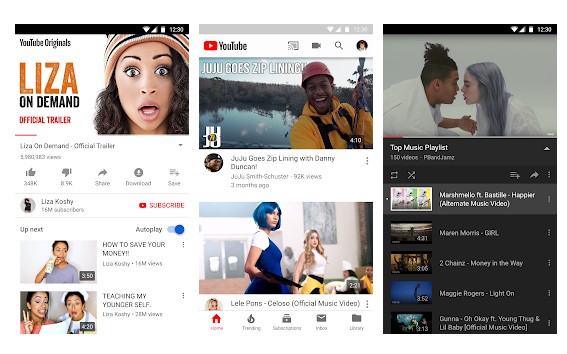The image depicts a website layout divided into three sections, each designed to resemble a separate smartphone screen. Here is a detailed description of each section:

**Top Section:**
- **Background:** Black
- **Status Bar:** Displays cell phone signal strength, Wi-Fi signal, battery level, and the time, which is 12:30.
- **Content:**
  - Title: "YouTube Originals: Lies on Demand Official Trailer" (with "Official Trailer" in red and a red line underneath it).
  - Additional Text: "Lies on Demand Official Trailer."
  - Views: The number of views is blurry.
  - Engagements: "343K likes, 84K dislikes."
  - Sharing Options: "Share, Download, See."
  - Author Information: "By Liza Koshy," total subscriber count "16M subscribers."
  - Call to Action: "YouTube Subscribe" in red.
  - Up Next: "Auto plays on. Teaching my younger self."

**Middle Section:**
- **Background:** Medium grey
- **Status Bar:** Similar to the top section, showing time, signal strength, Wi-Fi, and battery level.
- **Content:**
  - Header: "YouTube"
  - Featured Video: "JuJu Goes Zip Lining with Danny Duncan."
  - Additional Video: "Lele Pons: So So Official Music Video."

**Bottom Section:**
- **Background:** Black
- **Status Bar:** Similar to the other sections.
- **Content:**
  - Images: Shows two individuals.
  - Playlist Title: "Top Music Playlist"
  - Featured Songs:
    1. "Marshmello featuring Bastille - Happier"
    2. "Maren Morris - 2 Chainz"
    3. "Maggie Rogers - Quanah" (featuring Young Thug).

This organized and detailed caption provides a comprehensive understanding of the website layout and its contents.